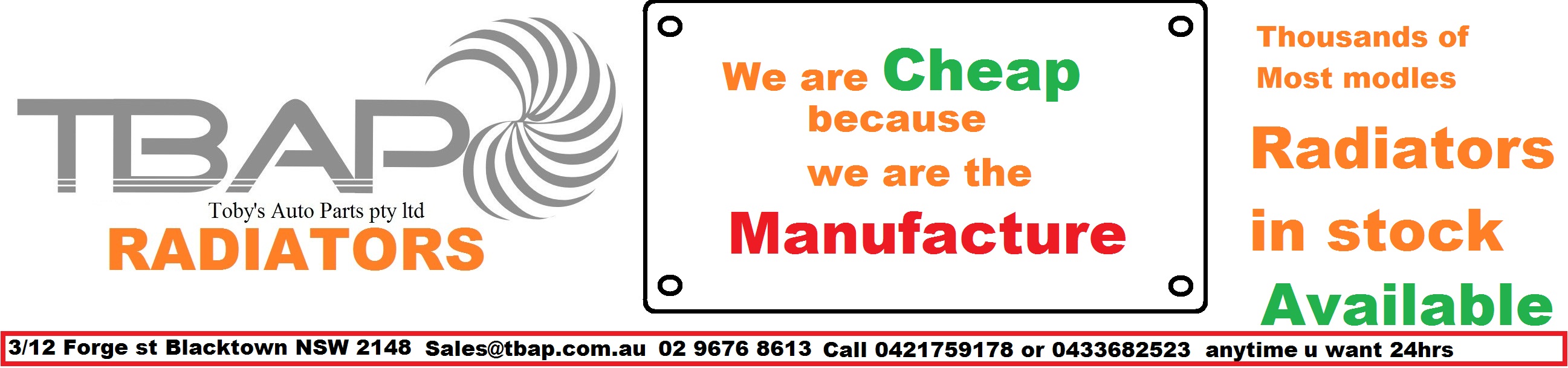This rectangular advertisement, wider than it is tall, predominantly features a central design resembling a license plate with four fastening holes in the corners. At the top left, in bold gray letters with a spiral pattern, it reads "T-BAP," indicating Toby's Auto Parts Pty Limited, followed by "Radiators." Below this, an orange text section states "We Are," followed by the green text "Cheap," and orange text again "Because We Are The," finishing with a red "Manufacturer." Adjacent to this, in small orange writing, it reads "Thousands of most models radiators in stock," with "available" highlighted in green below. The bottom section, outlined in red, provides contact details: "3-12 Forge Street, Blacktown, NSW 2148," the email "sales@tbap.com.au," and phone numbers "02-9676-8613," "042-1759-178," and "0433-682523," available "anytime you want, 24 hours." The letter "U" is used uniquely in place of "you."